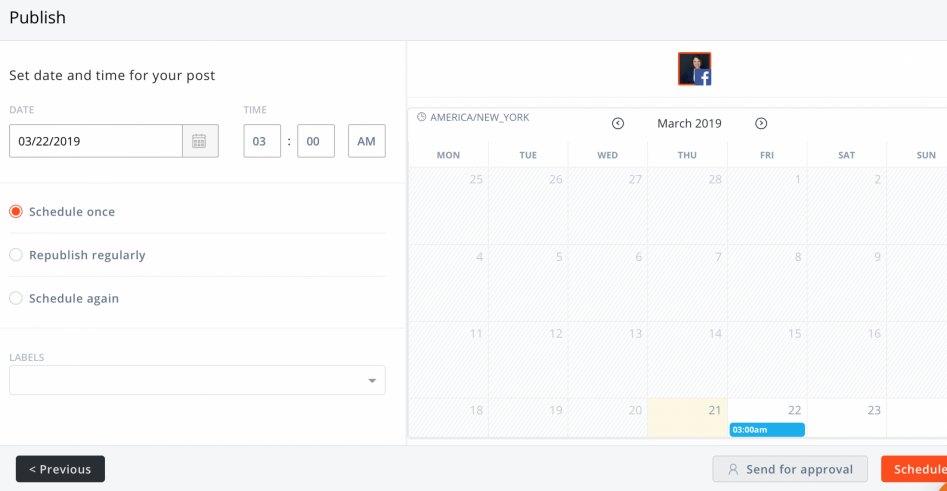Screenshot of a Social Media Post Scheduling Tool Interface

This image appears to be a screenshot from a web page or application designed to schedule social media posts. At the top of the screen, there's a prominent heading that reads "Publish." Directly below this, there is an instruction to "Set date and time for your post," accompanied by a drop-down menu that displays a calendar. The currently selected date is March 22, 2019, noted as "03-22-2019," with the time set to 3:00 AM ("03:00 AM").

The interface offers several scheduling options: 
1. "Schedule once" – which is selected via a radio button.
2. "Republish regularly" 
3. "Schedule again."

Under these options, there's a section labeled "Add labels," which is currently empty. Moving further down, there's a button labeled "Previous," allowing users to navigate back to the previous page.

To the right side of the image, there's a thumbnail-sized picture with a small Facebook logo in its corner, suggesting that the post is intended for Facebook. This section also provides an expanded view of the calendar, clearly highlighting the selected date.

Below the calendar, two buttons are available:
1. "Send for approval," featuring an icon of a generic person.
2. An orange button labeled "Schedule."

The overall layout of the screenshot indicates that it is in landscape orientation, suggesting the interface is designed for use on a desktop computer rather than a smartphone.